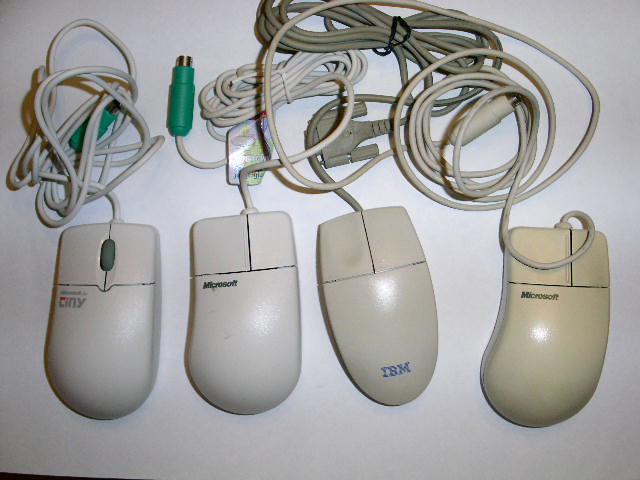The photograph showcases a collection of four vintage computer mice arranged horizontally on a plain white surface. Each mouse, varying in shades from white to yellowed beige, is accompanied by a coiled cable positioned above them. 

Starting from the left, the first mouse is a grayish-white, squared towards the top with a dark gray roller and an indistinguishable brand name on the top left palm section. This mouse features a PS2 connector with a green base. Next, we have a Microsoft-branded mouse, more curved on the left side and without a middle button. It also has a PS2 connector with a green base, mirroring the connectivity of the first mouse.

The third mouse is a beige IBM model, unique for its blue IBM branding at the bottom center and an oval end shape. This mouse is connected via a VGA connector, indicating its considerable age. Lastly, on the far right, there’s another Microsoft mouse, identical in design to the second but significantly yellowed with time. This one too connects via a PS2 port.

Overall, this collection, likely from the early or late 90s, presents an interesting snapshot of historical computer peripherals.